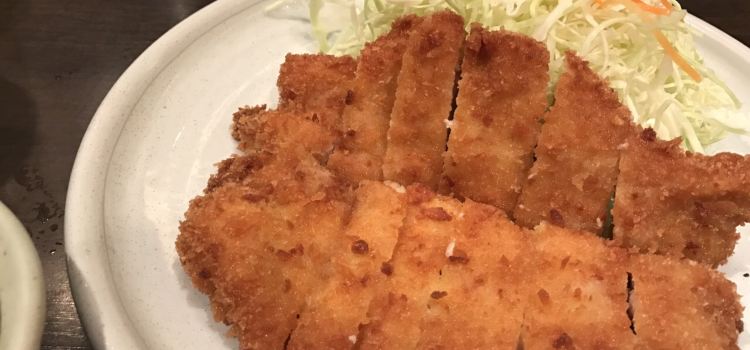This image showcases a beautifully plated dish of fried food, either fish or chicken, sliced into thin, narrow strips and perfectly breaded to a golden brown crisp. The food is elegantly arranged atop a cream-colored, ceramic plate with raised lips, and is accompanied by a vibrant portion of coleslaw or possibly thinly sliced vegetables that include green, white, and orange hues—indicative of lettuce or cabbage and shredded carrots. This plate rests on a dark brown table, photographed from a top-down perspective, capturing the indoor setting. A few water droplets are visible on the table to the left of the plate, adding a touch of realism to the scene. Adding to the composition, a fragment of another plate or bowl, of the same off-white stoneware, peeks in from the far-left bottom corner of the frame. The setting is devoid of any text or wording, leaving the focus solely on the visually appealing meal. With its meticulous presentation and balanced colors, this dish appears to be the highlight of a warm, inviting dining experience.